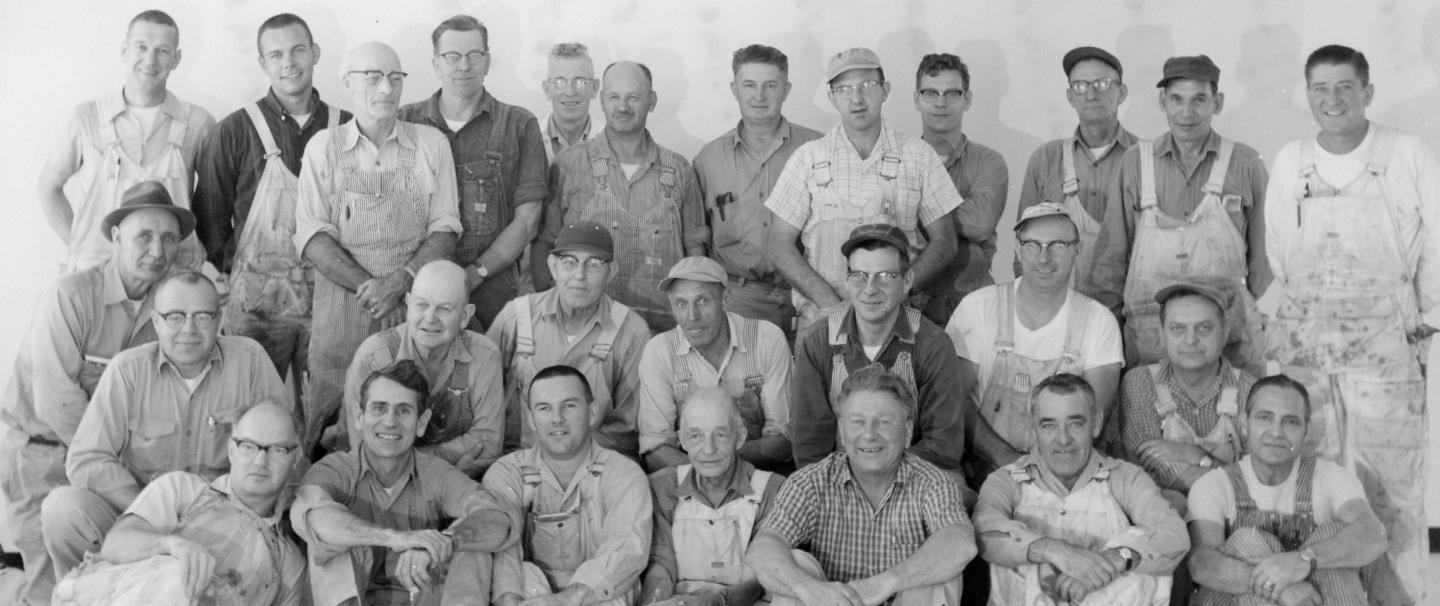This is an old black-and-white photograph of a group of approximately 40 white men, likely workers, arranged in three distinct rows in front of a plain gray wall. The front row consists of men sitting low to the ground, the middle row features men kneeling, and the back row has men standing. Most of the men are dressed in workwear, such as painter's pants, overalls, and tops that resemble smocks, implying they might belong to a painting or some other labor-intensive company. A man in a striped shirt seated at the front is smiling, possibly indicating a position of leadership or ownership, while another man wearing a hat and a collared shirt could be a supervisor. The photograph captures shadows of the men's heads on the wall behind them, adding depth to the image. The men's ages vary, although they appear older, with different styles of hats and shirts adding a variety of details to their ensemble.